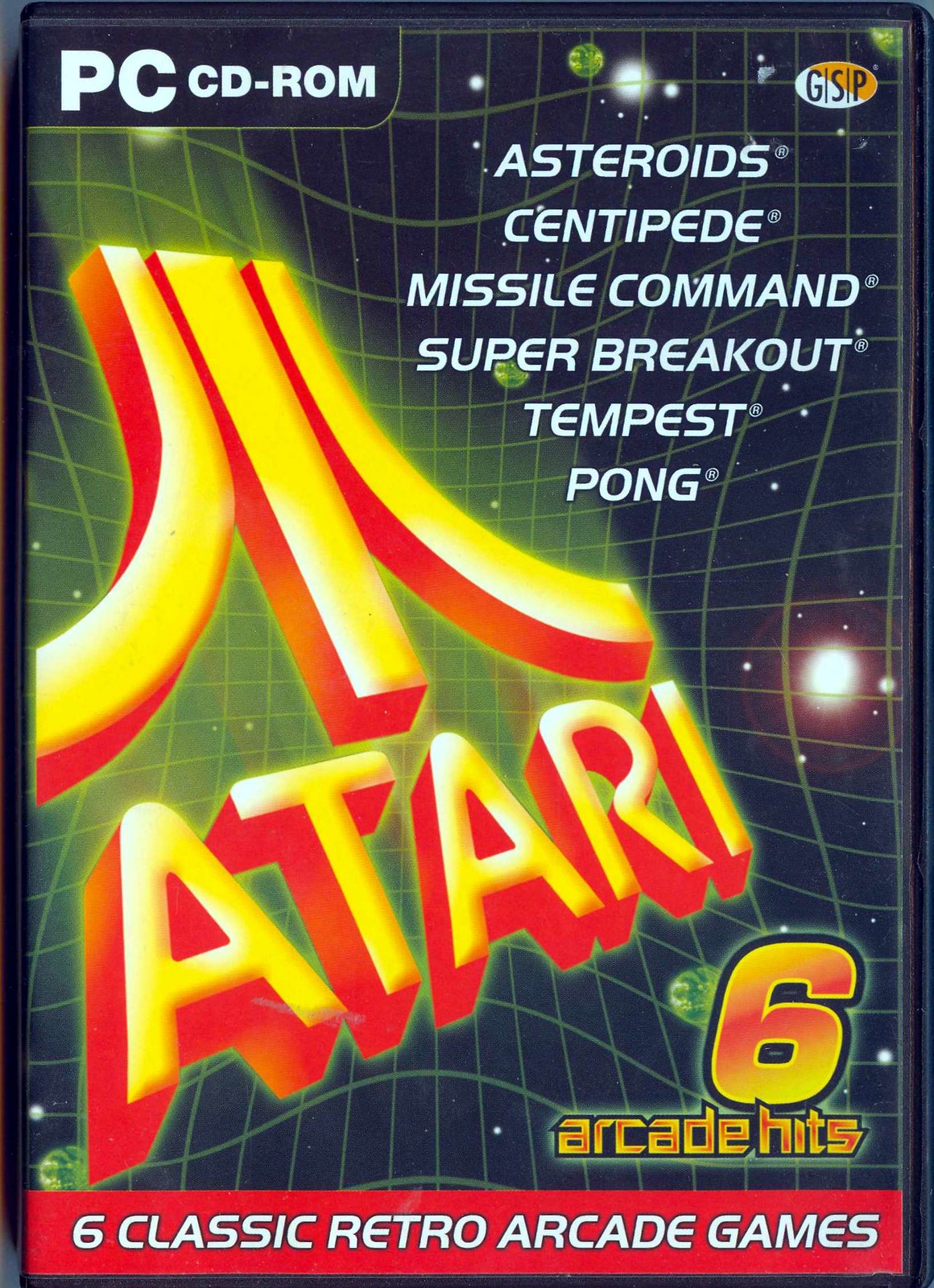This image depicts the box art for a compilation of classic Atari video games. The cover is primarily black with a slightly distorted, light green grid and small lights possibly representing planets. In the top left corner, the white text reads "PC CD-ROM," indicating the platform. 

On the top right, there's a white and orange logo with the text "GSP" in black. Directly below, in white text, the included games are listed: "Asteroids, Centipede, Missile Command, Super Breakout, Tempest, Pong." 

On the left side, a prominent yellow and red Atari logo is situated with the word "Atari" beneath it. In the bottom right, a red and yellow "6" is displayed, underlined by the caption "Arcade Hits." Along the bottom of the cover, a horizontal red bar contains white text with black trim stating "6 Classic Retro Arcade Games," emphasizing the compilation nature of the product.